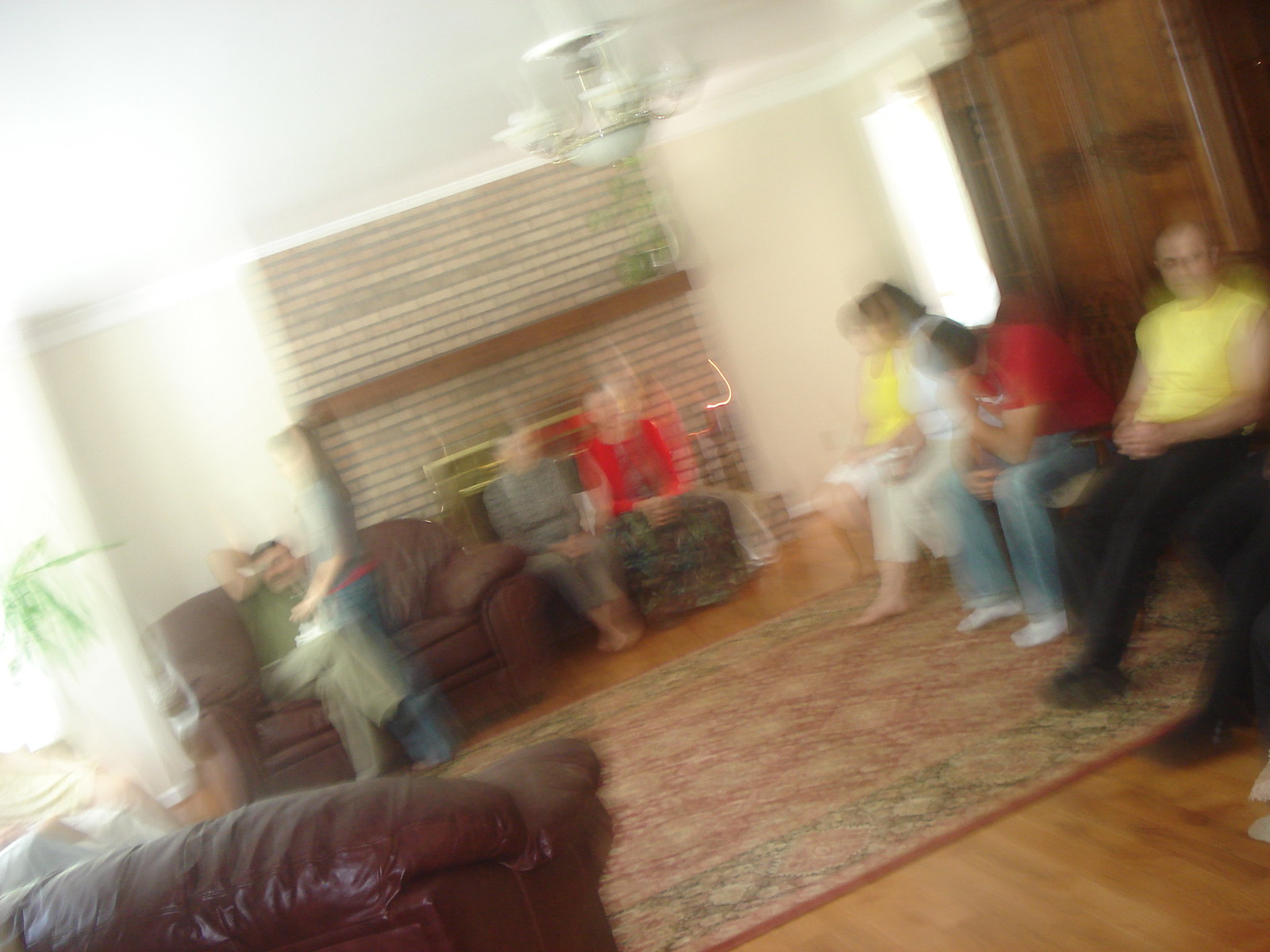In a blurry and slanted image of a living room, a gathering of people appears to be in discussion or making decisions. The room features a hardwood floor and an oriental rug in the center, along with several leather furniture pieces. Along the left side, a brown leather loveseat seats a man whose distorted arm seems AI-generated, reflecting the image's blur. In front of a fireplace at the far end of the room, which slightly tilts towards the right, two individuals—a man and a woman—sit on the hearth. There's a plant visible on the window ledge with light streaming in from a partially viewable window. A chair is also before the fireplace.

On the right-hand side, four more people, out of focus, are seated. Their outfits are somewhat discernible: one in a yellow shirt, another in red, one in white, and again, another in yellow. One person in a yellow shirt appears to be reading something aloud while a person in a red shirt listens intently with their head turned. Additionally, a person in a grey shirt and someone in denim can be seen on the left. The image, overall, conveys a sense of an informal gathering or meeting amidst a cozy, lived-in space.